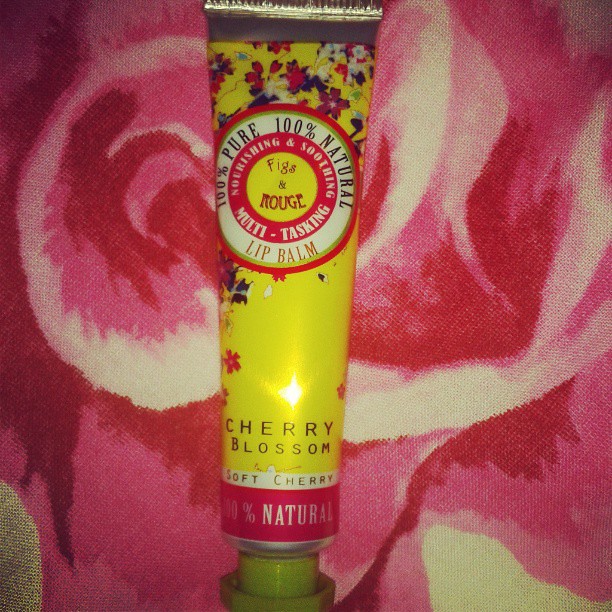The photograph displays a metal squeeze tube of lip balm by the brand Figs and Rouge, placed on a background with a rose print that could be a tablecloth or a towel. The predominantly yellow tube features a visually appealing design with cherry blossom flowers illustrated mainly on its upper half, cascading downwards. It has a beige-greenish screw-on cap. Prominently displayed on the tube is a circle with the text "100% pure, 100% natural," and within that circle, phrases like "nourishing and soothing" and "multitasking" are highlighted. The brand name, "Figs and Rouge," is also indicated. At the bottom portion of the tube, in dark text, the words "cherry blossom" are written, followed by a white banner stating "soft cherry" and a pink section noting "100% natural." The product description suggests it is a 100% natural cherry blossom-flavored or scented lip balm.